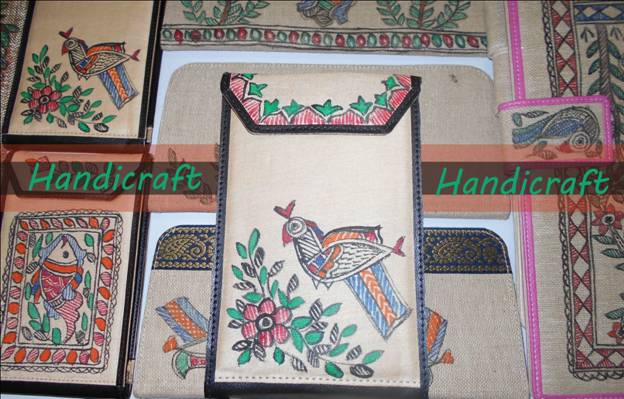A display of handcrafted pouches is spread out on a flat surface, possibly for sale. The pouches are cream-colored with black or colorful borders. The central pouch, rectangular and perhaps intended for glasses or other small items, features vibrant artwork, including a bird outlined in black with green and pink designs. Surrounding the bird are images of plants, flowers, and possibly fish, enriched with a palette of reds, oranges, greens, blues, and white. The flap of this pouch has triangular designs and hexagon shapes. Across the image, a semi-transparent black bar with bright green lettering spells "handicraft" on both the left and right sides, emphasizing the artisanal nature of these items. The background of the display is tan, adding to the traditional feel of the artwork.